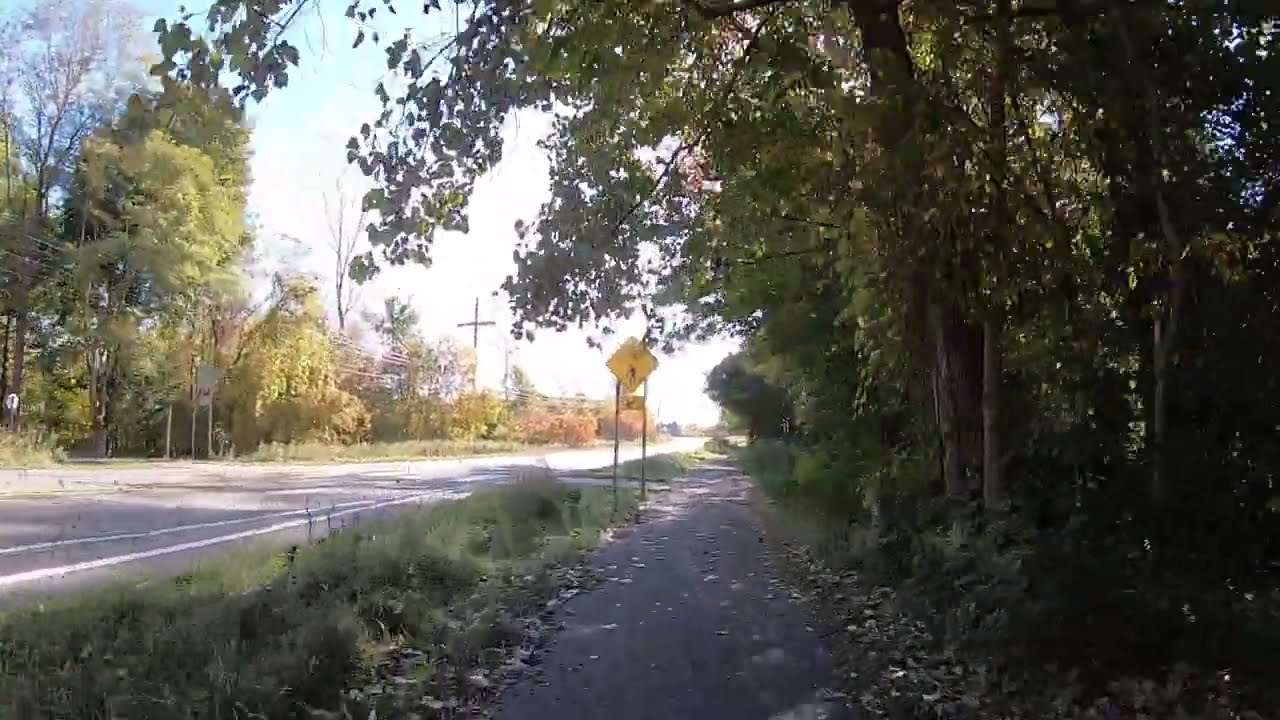The image features a gravel sidewalk running alongside an empty road, capturing a serene and natural setting. The sidewalk, possibly a walking or biking path, is bordered by dense greenery with leaves and plants scattered on the ground, indicating a rural or woodland area. Towering deciduous trees line both sides of the road, casting shadows over the deserted street, which appears to be a single, wide lane. In the center of the composition, a yellow street sign with a pedestrian symbol, supported by two poles, alerts drivers to the presence of walkers. The road and the sidewalk stretch straight into the distance, under the bright midday sun with clear skies overhead. In the far background, a structure resembling a wire post, shaped like a cross, can be seen behind the trees, complementing the natural scenery.